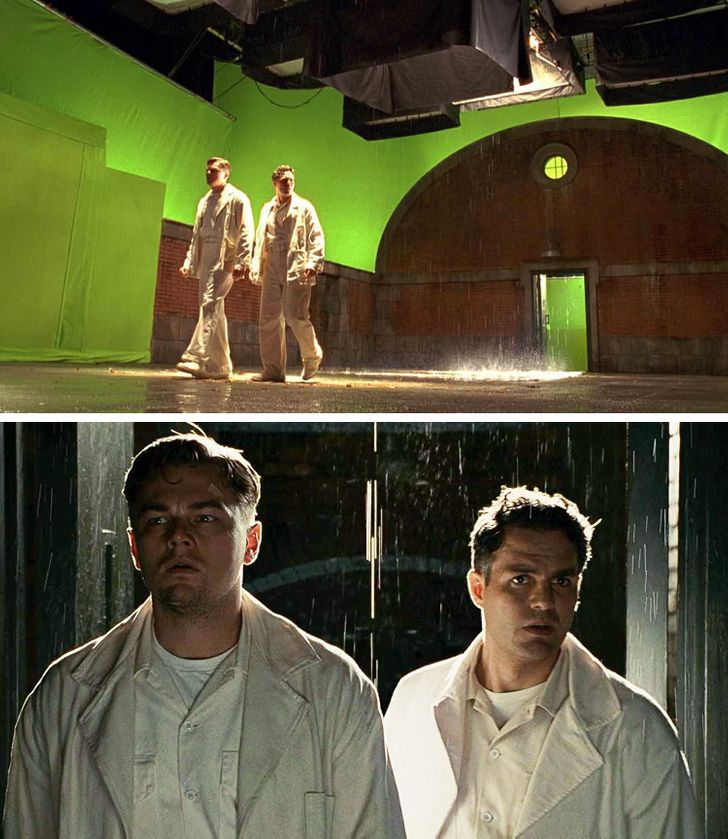The image consists of two rectangular still shots from a movie set. In the top panel, Leonardo DiCaprio and Mark Ruffalo, dressed in all-white outfits including jackets and pants, are seen walking towards the left side of the frame. The scene features prominent green screens and sophisticated studio lighting equipment hanging from the ceiling, likely used for special effects. A brown arched doorway and wall are also visible in the background, indicating the set design.

The bottom panel offers a close-up of DiCaprio and Ruffalo, which appears to be a final edited shot from the movie. DiCaprio, on the left, shows a forlorn expression while wearing a white t-shirt under a white button-up and jacket. Ruffalo, on the right, dressed similarly to DiCaprio, has a quizzical look and faces slightly to the right. Behind them, through the arched doorway, it is dark and rainy, with light sources illuminating their heads and faces, enhancing the dramatic atmosphere of the scene.